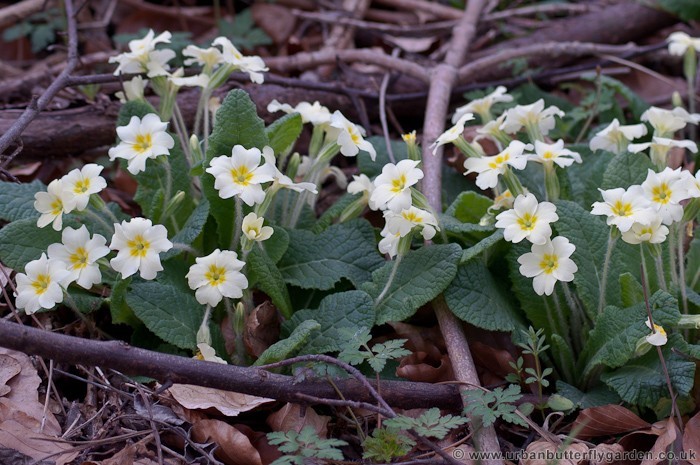The photograph captures a detailed and vibrant scene of a forest floor, featuring an array of wildflowers amidst natural debris. The ground is littered with dead leaves, sticks, and twigs, providing a rich, rustic backdrop for the blooming flora. Prominently in the bottom right, marked with a copyright watermark from www.urbanbutterflygarden.co.uk, we observe a flowering plant with slender, dark and light branches that extend upward and across the frame. The plant boasts oval green leaves with pronounced veins and deep texture, while the flowers themselves are primarily white with five forked petals circling a yellow center. At the very heart of each flower, a green stamen is visible. These wildflowers, possibly wild primroses, are abundant, with several clusters oriented in various directions. Additionally, a more delicate, fern-like plant appears in the foreground, adding to the lush diversity of this natural scene.